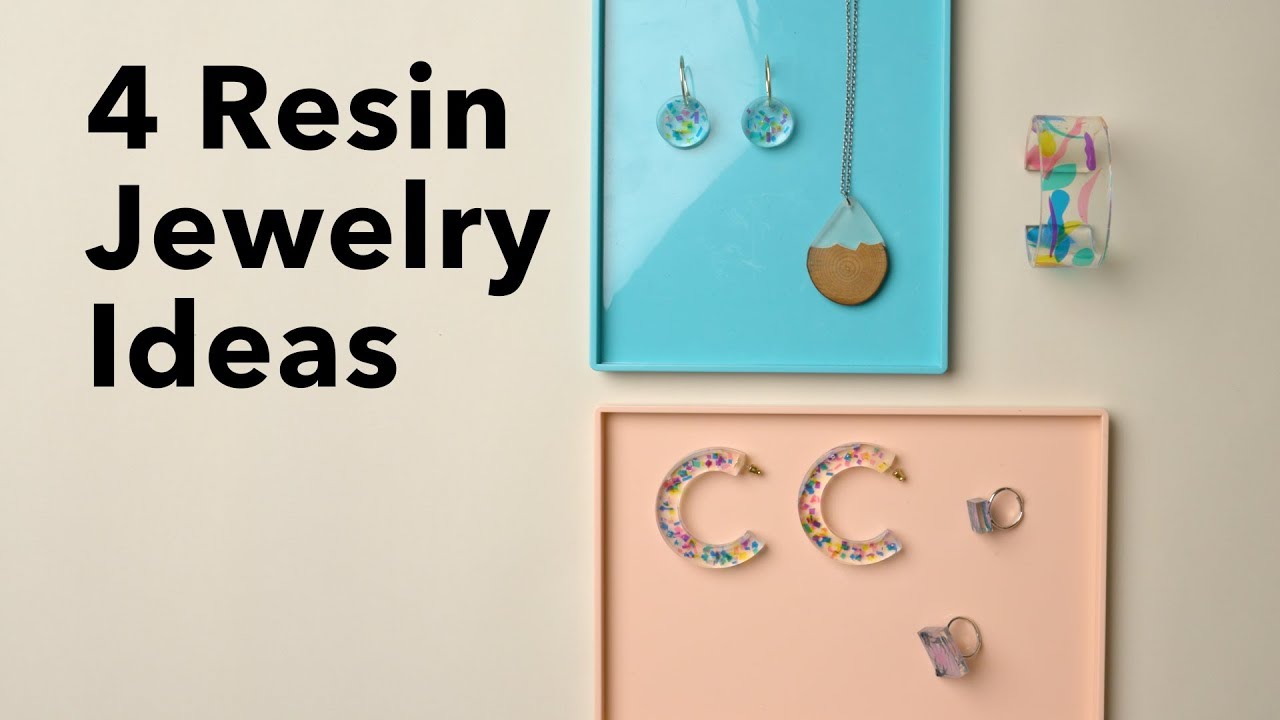This image showcases an artistic assortment of resin jewelry, reminiscent of something you might find on a Pinterest board. Presented against a black background, the text reads "Four Resin Jewelry Ideas," though the display actually features six distinct pieces. 

At the top, a vibrant bangle bracelet is adorned with an array of colorful paint smudges—purple, pink, blue, green, and yellow—viewed from a top-down perspective. Beneath this, a blue frame contains two circular resin earrings, each embellished with multicolored splotches of yellow, blue, pink, purple, and green. 

Also within the blue frame is a necklace with a teardrop-shaped pendant; its upper section is a delicate pale blue, transitioning into a wood-like brown hue at the base, and it is suspended on a silver chain. 

The bottom section of the image features a pale pink frame displaying two translucent resin hoop earrings, arranged in a 'C' shape and decorated with varied paint splotches of green, red, pink, blue, and purple. Accompanying these are two finger rings, slightly differing in size, both rendered in a pale purple, glass-like, transparent resin.

Together, these pieces highlight several creative and colorful resin jewelry ideas, showcasing the versatile beauty of resin as a medium.